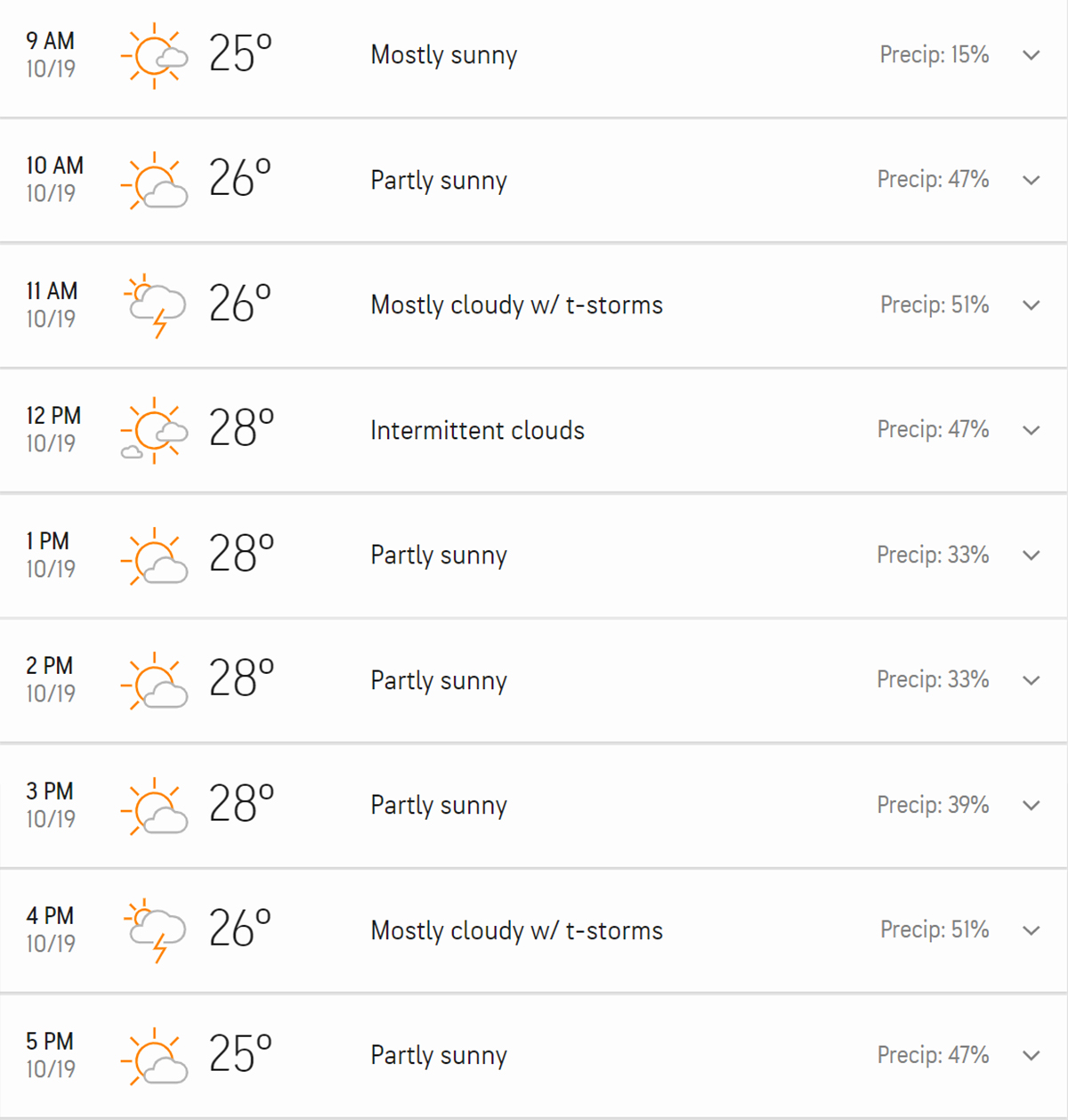The image features a detailed weather forecast displayed against a stark white background. The majority of the text is in black or gray fonts, providing clear contrast for readability. The weather icons include an orange sun and a gray-outlined cloud, representing different weather conditions. 

The forecast focuses on October 19th, showing hourly predictions:

- **9 a.m.:** The temperature will be 25 degrees (likely in Fahrenheit). The weather will be mostly sunny with a precipitation probability of 15%.
- **10 a.m.:** The temperature will rise slightly to 26 degrees, with partly sunny skies and a 47% chance of precipitation.
- **11 a.m.:** The temperature remains 26 degrees but shifts to mostly cloudy conditions with thunderstorms expected. The chance of precipitation increases to 51%.
- **12 p.m.:** The temperature reaches 28 degrees, with intermittent clouds and a 47% probability of precipitation.

The forecast focuses on fluctuations in cloud cover and precipitation predictions throughout the late morning to midday hours.